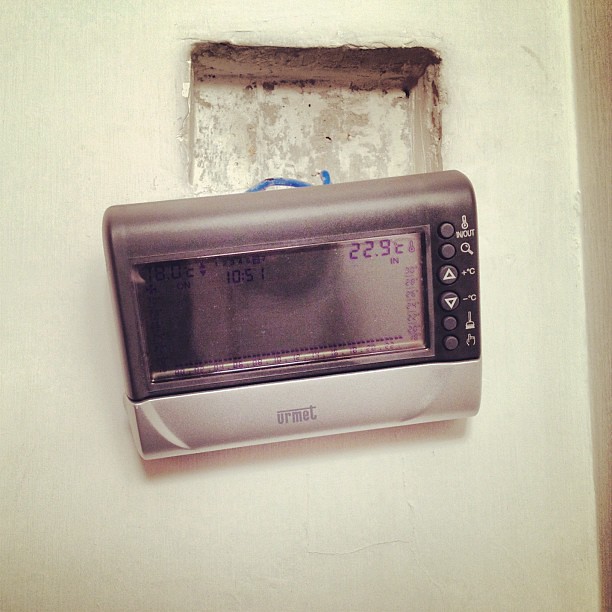In this detailed photograph, a temperature control device has come loose from its casing embedded in a rough-textured, grainy white wall. The device, oriented horizontally, has a predominantly black upper section with a white base. The black portion occupies about 80% of the device's surface area and features a dark screen displaying blue-hued figures, including the numbers 18.0, 1051, and 22.9°C. Adjacent to the screen are several black buttons with white labels. The labels include "In-Out," a magnifying glass icon, up and down arrows accompanied by plus and minus Celsius symbols, a paintbrush icon, and an icon depicting a hand. The white base prominently displays the branding "You Are Met." The device is precariously hanging from a hole in the wall, connected by a blue wire, suggesting that it might have fallen out of its mounting. This device is likely used for temperature control.